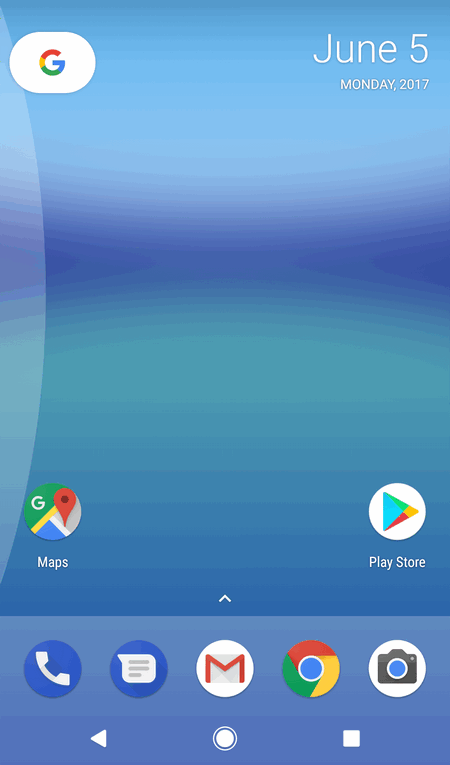In the image displayed on the computer screen, the upper left corner features the iconic Google logo, characterized by a capital 'G' adorned in red, yellow, green, and blue colors. Adjacent to the logo on the right, the date is prominently displayed as "June 5th, Monday, 2017". The background of the screen is a soothing wavy blue pattern, adding a dynamic visual texture.

Centrally located is the Google Maps icon, depicted as a circular icon combining green, blue, and yellow segments with a distinctive red pin marker. Adjacent to this is the Google Play Store icon. Down towards the bottom of the screen, there are several interactive buttons. On the far left, a call button is visibly positioned. To its right, there is a chat button situated in the middle of the row. Next in line is the mail button, easily identifiable by an envelope symbol with an 'M' inside it. 

Towards the right side of the screen, another Google icon is present, exhibiting the familiar red, green, yellow, and blue colors. Lastly, a camera icon is also visible, completing the array of function buttons displayed on the screen.